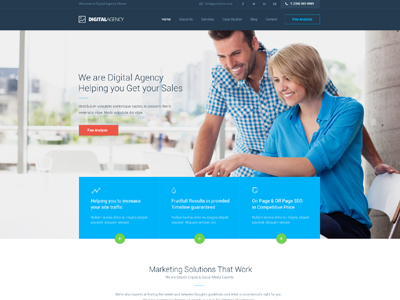This slightly blurry screenshot depicts the homepage of a Digital Agency. The website banner proudly states, "We are Digital Agency, helping you get your sales." Directly below, the details remain indistinct, but it features a bold red box, presumably a call-to-action button, alongside a blue box with three green circles beneath it.

The layout consists of three main sections. The first section seems to focus on driving traffic results, although the exact wording is not clear. The second section also mentions results, but specifics are illegible. The third section appears to discuss page optimization, but key text is too blurry to decipher.

Accompanying these sections is an image of a man and woman, both dressed in shades of blue. The man sports a blue checkered shirt, short brown hair, and a subtle five o'clock shadow. The woman has blonde hair styled in a bob and wears a solid blue shirt. They both smile warmly, showcasing their teeth. The man casually rests his left hand on the back of the woman's chair, as she leans forward and points at the screen of a white laptop on a white table between them. Behind them, a cityscape with high rises, trees, and a bannister populated with blurry figures is visible.

Below the three green circles, the text reads "Marketing solutions that work," but the finer print remains unreadable despite enlarging the image as it only increases the blurriness.